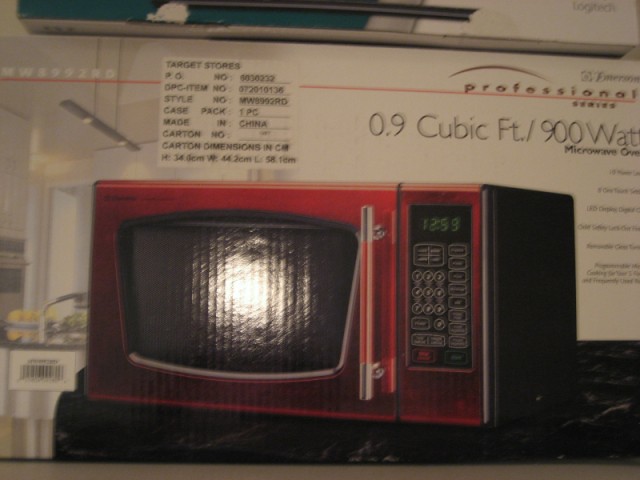The image captures a display of a half black, half red Emerson microwave at a Target store. The microwave is relatively small, with a capacity of 0.9 cubic feet and a power output of 900 watts. Its door features a unique design with the top portion in red, gradually fading into black at the bottom. The door handle is gray at the tips and transitions to red in the center. The microwave's control panel, located on the right, displays buttons numbered 1 through 9 and 0, along with various other function buttons. The LED clock reads 12:59 in green against a black background. The box, partially visible behind the microwave, echoes the details with the professional series branding and similar specifications. The box itself is white, with a Target Stores sticker indicating its retail location. A glare and slight out-of-focus quality obscure parts of the box's text.